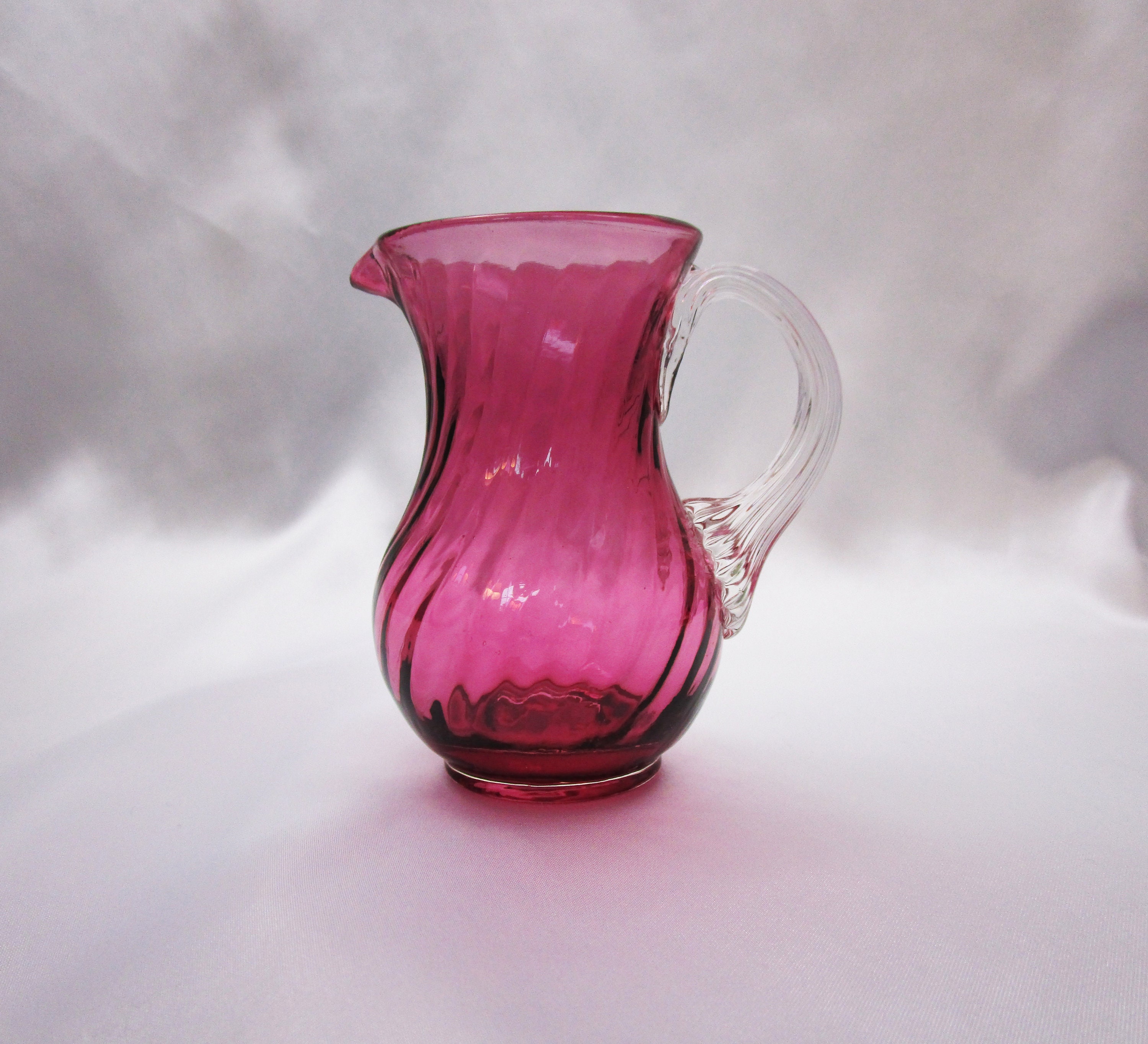The image displays a small, hand-blown cranberry glass pitcher, prominently centered against a misty, cloud-like backdrop of whites and grays. The pitcher itself exhibits a captivating swirl pattern in the glass, transitioning from a darker pink at the bottom to a lighter, almost rosy hue as it rises. This swirl continues elegantly into the clear glass handle, which is thinner at the top and thickens towards the bottom, providing a sturdy grip. The pitcher features a rolled rim at the top with a spout positioned on the left, opposite the handle. The bottom of the pitcher is also rolled, providing a flat base for stability. Despite its new appearance, the style suggests an antique quality, making it a likely display piece rather than a functional item. The overall presentation, with its vivid contrast against the soft background, makes it aesthetically striking and suggests it could be an advertisement or a listing photo for a vintage item on platforms like eBay or Mercari.